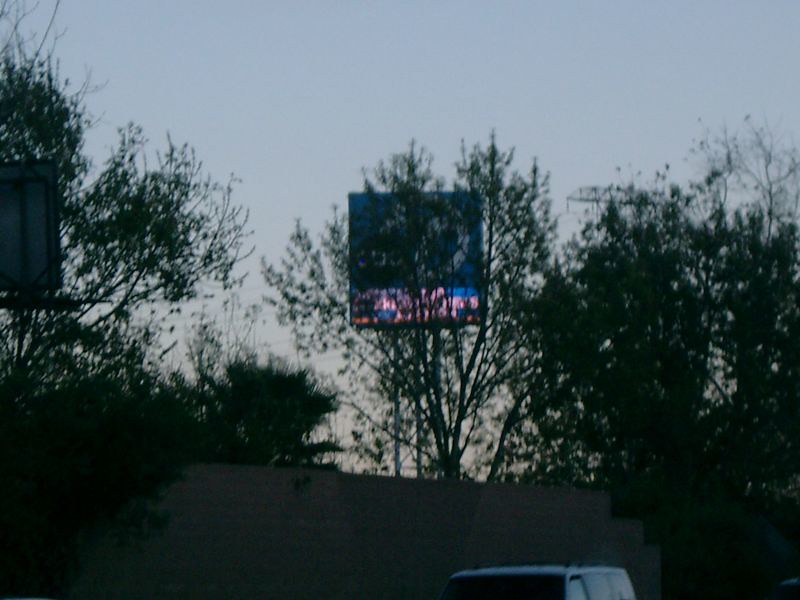Under a moody gray sky, a sparse cluster of trees partially obscures a dark gray-roofed house. A white van is parked adjacent to the house. To the left, the back of a sign is visible, while a large, illuminated blue sign with white text stands among the trees. The sign's bottom section transitions to blue with pink text and is near a light pole. The scene is enveloped in a mix of grays, with scattered trees and the presence of the white van adding to the overall somber ambiance.